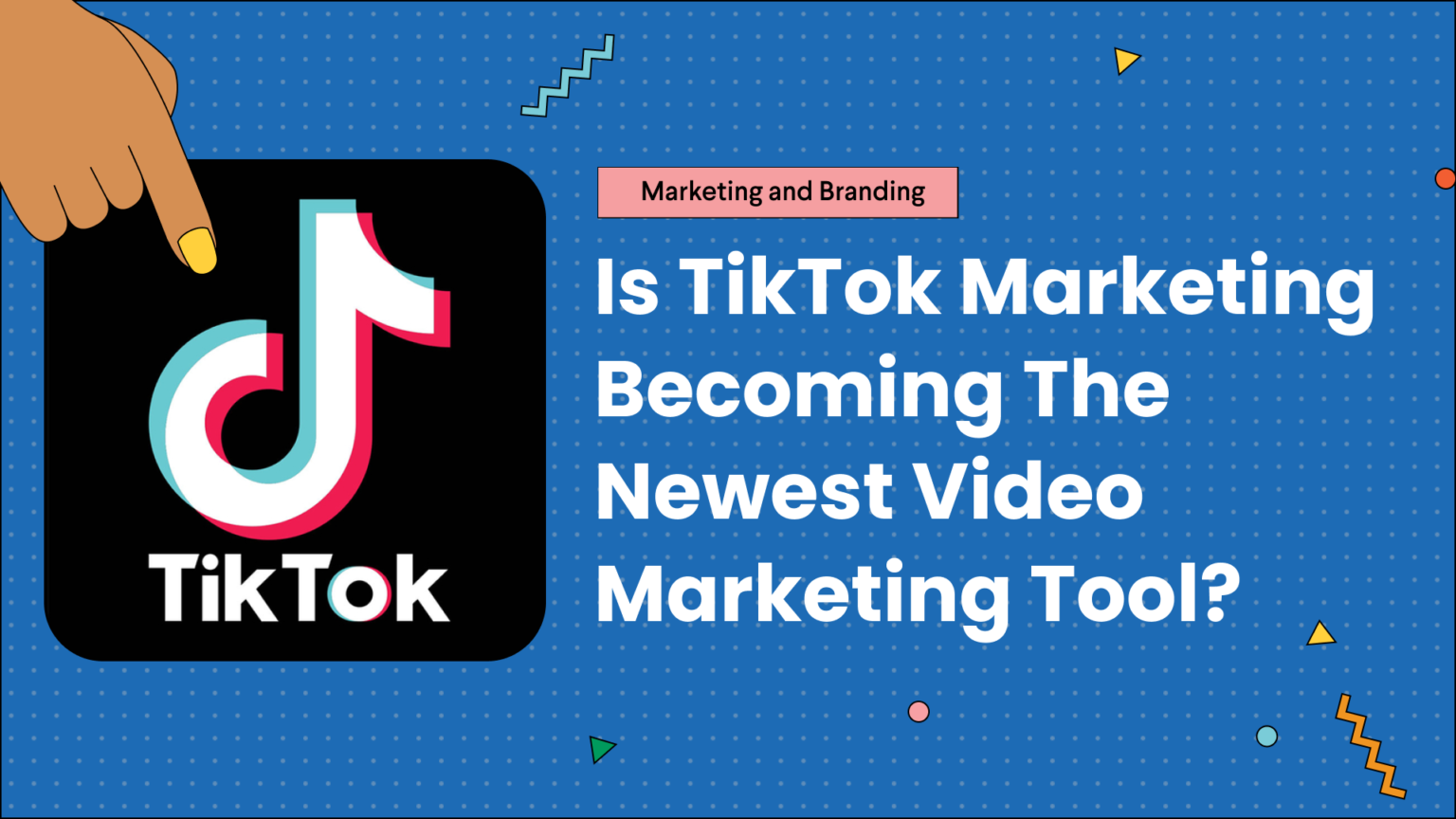This image is a promotional ad for TikTok, featuring a visually engaging and detailed design. The background is a deep blue dotted with rows of tiny white dots, creating a starry-like effect. On the left side, the prominent TikTok icon is displayed, encapsulating its profile. The icon features a black background with the recognizable TikTok logo—a stylized "T" in hues of blue, white, and red—with 'TikTok' written underneath in white. A brown hand with a yellow nail is pointing directly at the TikTok icon, drawing immediate attention to it.

To the right of the TikTok icon is a vibrant pink banner with black text that reads "Marketing and Branding." Beneath this, in white text, the banner poses the question: "Is TikTok marketing becoming the newest video marketing tool?" The question is emphasized with a question mark to intrigue the viewer.

The image is further adorned with scattered colored dots and geometric shapes, adding a playful touch. Notably, there are pink, blue, and red circular dots dispersed around the ad. Additional decorative elements include three triangular shapes—two in yellow and one in green. Complementing these are two squiggly lines, one in light teal and the other in orange, with the latter positioned at the bottom right corner of the image.

Overall, the ad blends vibrant colors, dynamic shapes, and intriguing text to effectively capture the viewer’s attention and convey the message.